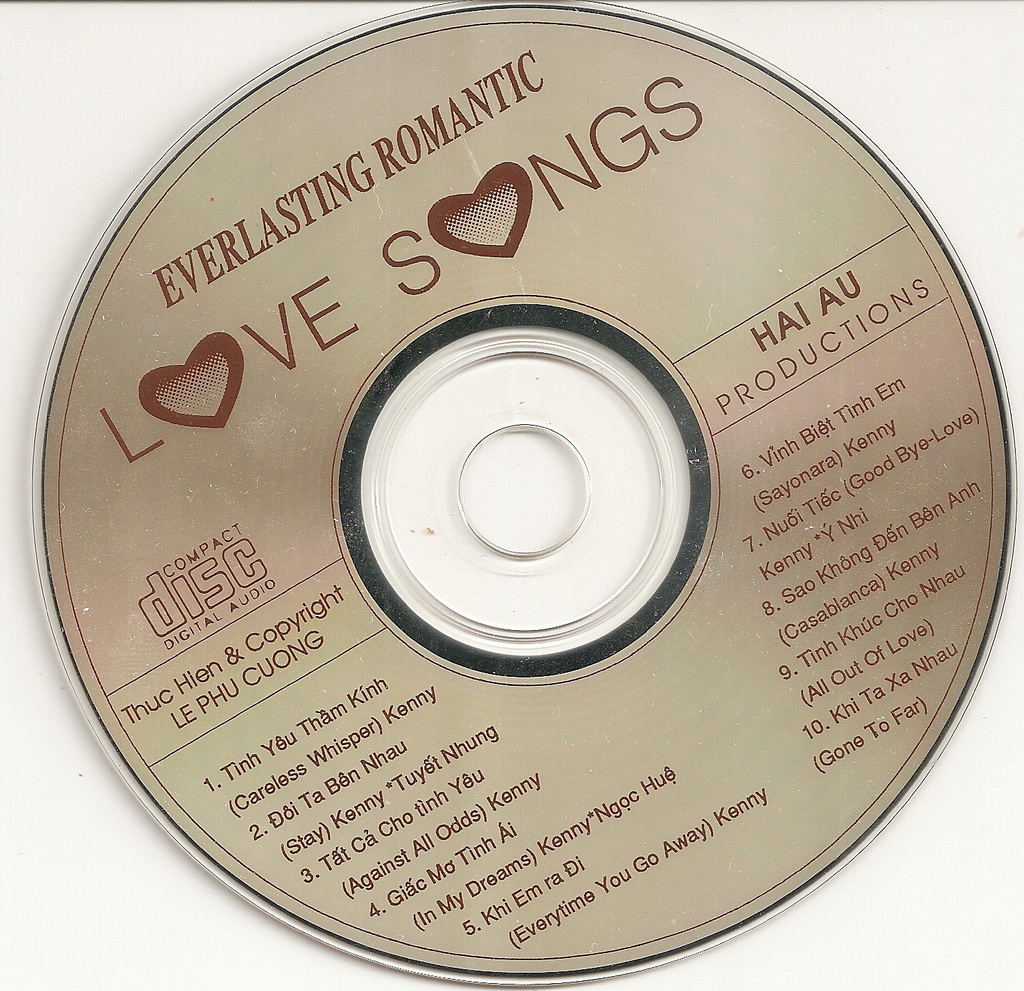The image depicts a CD titled "Everlasting Romantic Love Songs," featuring a tan background with faded brownish-red hues and a black rim surrounding the transparent center hole. The text on the CD is prominently displayed in red. At the top left in all capital letters, it reads "Everlasting Romantic," and below that, also in capital letters, it says "Love Songs," with hearts replacing the "O" in both words. Along the right side, the inscriptions include "Compact Disc Digital Audio," "Thuc Hynh," "Copyright Lei-Fu Chung," and "Hai-Ao Productions." The tracklist, featuring ten songs in both English and Vietnamese, is positioned below these details. The disc takes up the entire image, presenting a visual style that accentuates the text and design elements on its surface.